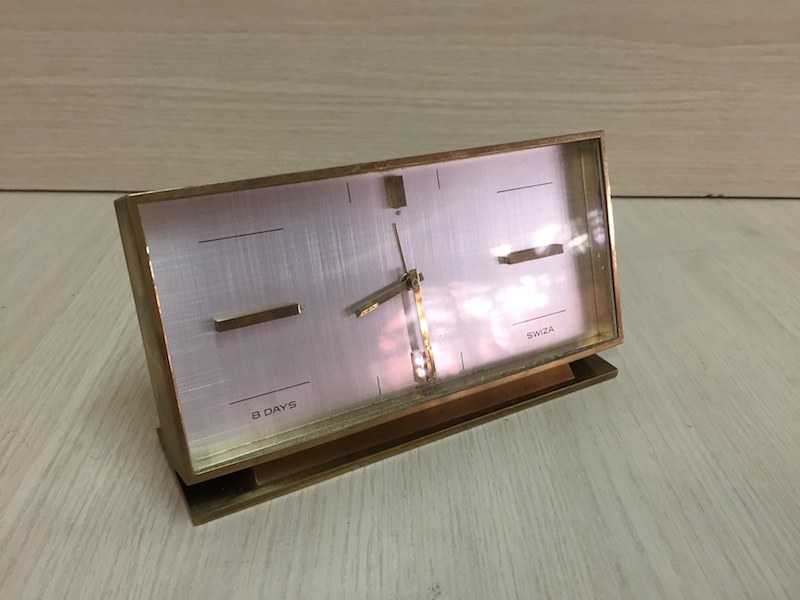This color photograph captures a vintage, state-of-the-art desk clock from the 1950s or 1960s, exhibiting a combination of an old-world aesthetic with a touch of mid-century modern design. The clock, diagonally oriented from the lower left to the upper right, sits on a taupe-colored tabletop that resembles either birchwood or formica. Its rectangular body features a striking framing made of gold or copper-colored metal, with a brushed silver dial face. The 12, 3, 6, and 9 positions are marked with bold dashes of matching metal, with faint markings indicating other time zones. The clock has three gold hands—the minute hand, the second hand, and the alarm-setting hand. Additionally, subtle inscriptions on the dial read "8 days" in the lower left corner and "Switzer" in the lower right. The entire unit is perched at a slight tilt on a flat, rectangular gold base, giving it an elegant yet nostalgic charm against the light wood-grained backdrop.